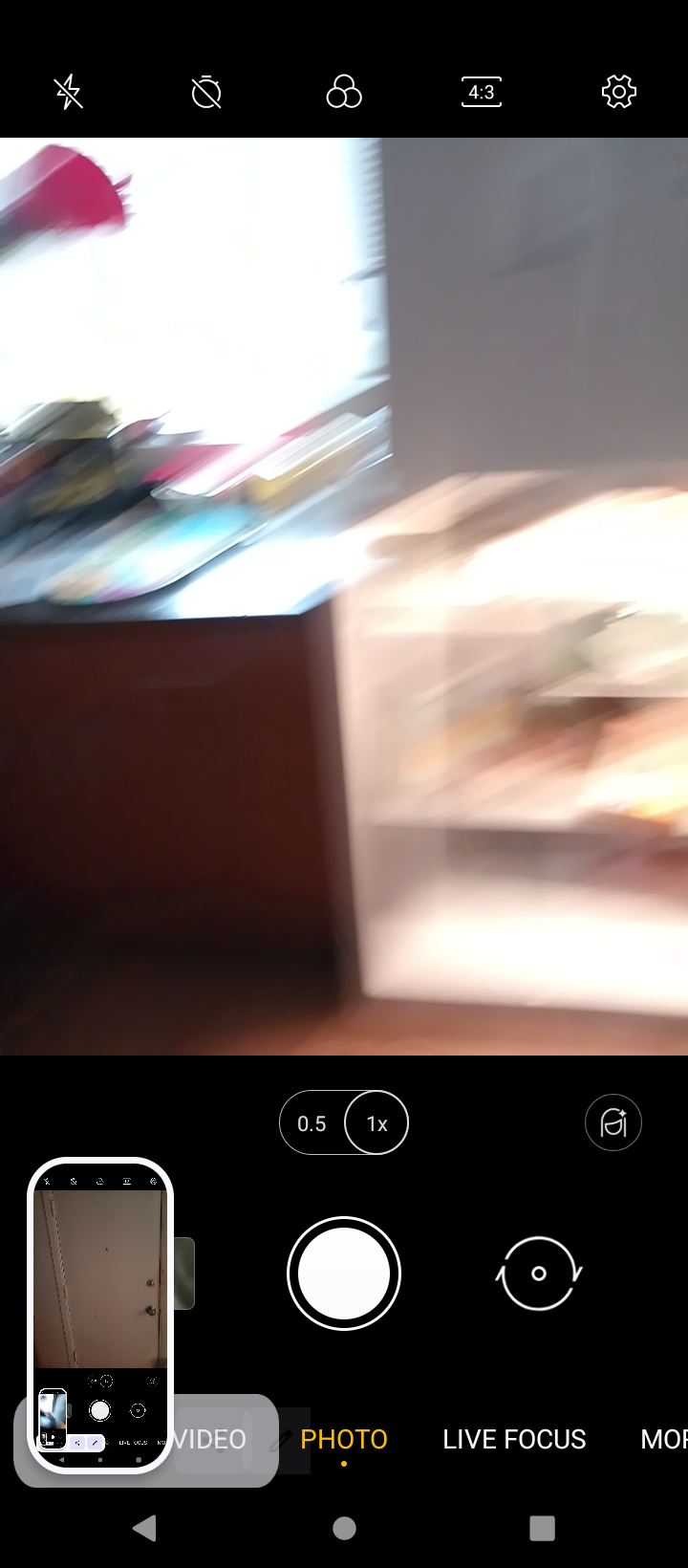**Caption:** 

A blurry cell phone photo capturing a cluttered desk space. The upper portion of the image features black bars with various icons—reminiscent of an active phone screen. Centrally, a hazy window sits above a desk that holds a small red lamp, a stack of books, and scattered papers. To the right of the desk, a white shelving unit crammed with more papers makes an appearance. The bottom part of the photo, encased in black, displays the phone's in-picture icons: a small phone image, "Photo" written in yellow, a large white shutter button, and other interface elements in black and light gray.